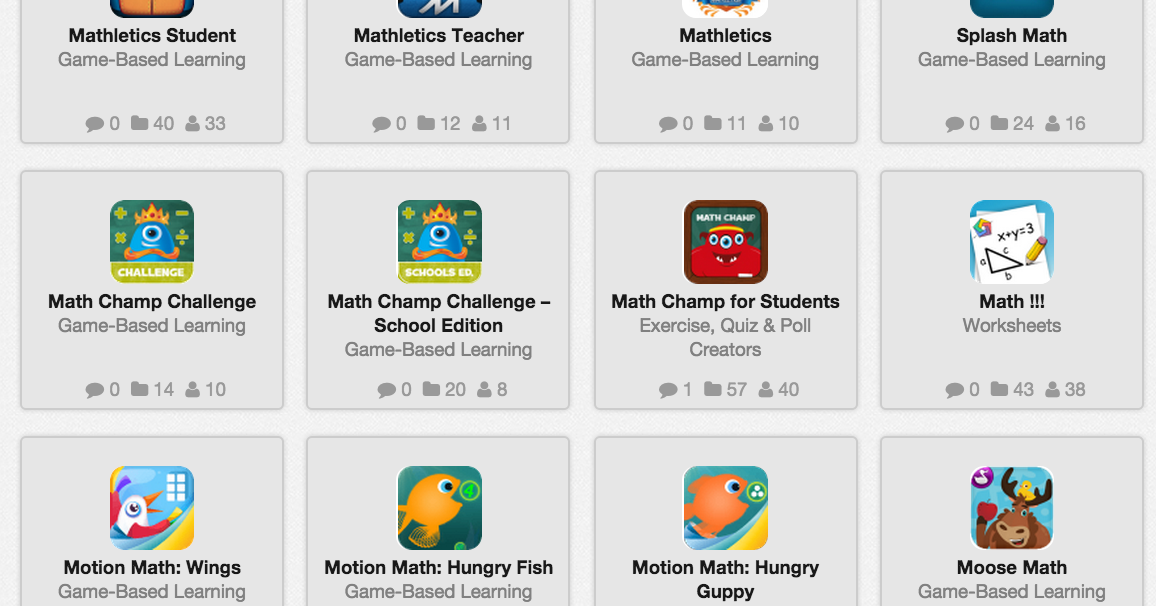The image depicts a third-party online app store specifically designed for educational purposes, with a focus on learning games for children. The app store features a variety of colorful app icons specifically aimed at young learners, likely ranging from first to sixth grade. These educational apps predominantly focus on enhancing math skills through interactive, game-based learning experiences. Notable apps include "Math Champ Challenge," "Math Champ School Edition," "Math Champ for Students," "Moose Math," "Motion Math Hungry Guppy," "Motion Math Hungry Fish," and "Motion Math Wings." Each app is designed to make math learning engaging and fun, allowing children to use tablets to practice and improve their math abilities through quizzes, exercises, and creative game play. This platform provides parents and educators with a valuable tool to support children's education through modern, intuitive, and enjoyable digital resources.